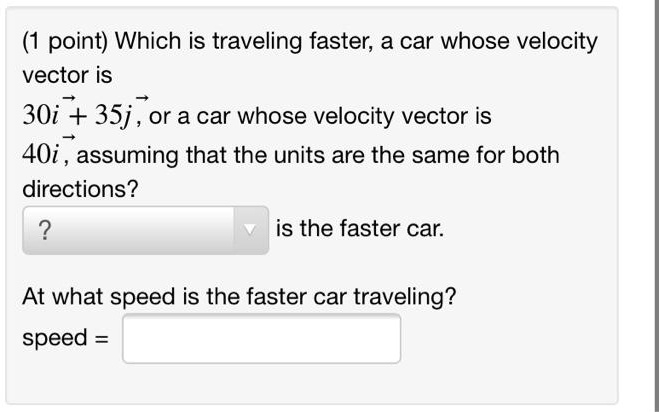The image features a gray background and presents a problem involving two cars traveling at different velocities. Car A has a velocity vector represented as \(30\hat{i} + 35\hat{j}\), while Car B has a velocity vector represented solely as \(40\hat{i}\). Both velocity vectors are depicted with rightward-pointing arrows. There's a rectangular box with a question mark in it, indicating the need to identify which car is faster. At the bottom, there is a prompt asking for the speed of the faster car, with "Speed =" followed by an empty box ready for the answer.